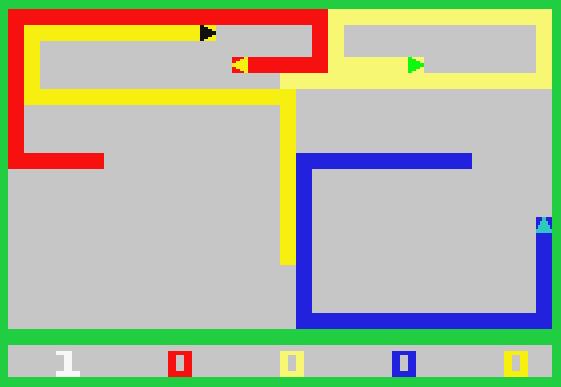The image features a gray background encased within a vibrant green border. Various colored lines—red, yellow, pale yellow, and blue—are scattered across the gray field, each with unique lengths and configurations. At the lower section of the image, a series of numbers are displayed: '1', '0', '0', '0', '0'. The '1' is depicted in white, the first '0' in red, the second '0' in yellow, the third '0' in blue, and the fourth '0' in bright yellow.

Interspersed among the lines are triangles that add an additional layer of complexity to the design. Each line harbors a distinctively colored triangle: a black triangle appears within the bright yellow line, a yellow triangle within the red line, a green triangle within the pale yellow line, and a turquoise triangle within the blue line. The careful arrangement and colorful elements create a visually striking, intricate composition.